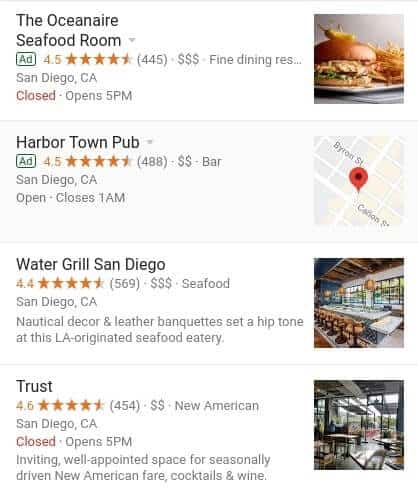The image showcases the search results for restaurants in San Diego, featuring four establishments with detailed information:

1. **Ocean Air Seafood Room:** 
    - Listed as an ad. 
    - Rated 4.5 stars with three dollar signs, indicating a pricey dining experience.
    - Categorized as a Fine Dining Restaurant.
    - Located in San Diego, California.
    - Currently closed, opens at 5 p.m.
    - Accompanied by a picture of a hamburger or sandwich with fries on the side.

2. **Harbortown Pub:**
    - Rated 4.5 stars with two dollar signs.
    - Located in San Diego, California.
    - Currently open, closes at 1 a.m.
    - Category: Bar.
    - Has a map image showing its location near Byron Street and Carlton Street (or Capon Street).

3. **Water Grill:**
    - Rated 4.4 stars with three dollar signs.
    - Located in San Diego, California.
    - Described as having nautical decor and leather banquettes, creating a hip atmosphere at this seafood eatery, originally from L.A.
    - Accompanied by an image of a long central table with swivel stools, surrounded by large windows.

4. **Trust:**
    - Rated 4.6 stars with two dollar signs.
    - Categorized as New American cuisine.
    - Located in San Diego, California.
    - Currently closed, opens at 5 p.m.
    - Described as an inviting, well-appointed space offering seasonally driven New American fare, cocktails, and wine.
    - The image shows a restaurant interior with glass windows and visible tables, though the picture is somewhat hard to decipher.

This detailed description succinctly presents the relevant information about each restaurant as shown in the search results.